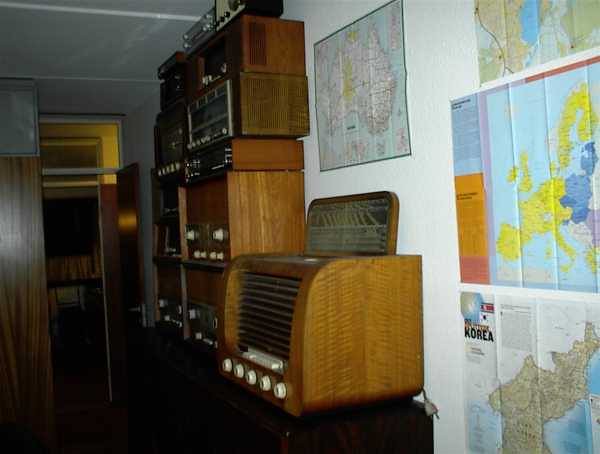The photograph is a full-color, somewhat dated indoor scene. Dominating the right side of the image are several maps, prominently featuring one vibrant in yellow, blue, and purple. Below it is a brown-hued map labeled "Korea," with additional maps that are less distinguishable. Among these additional maps, one appears to be of Europe and another of Australia. Arranged in a vertical sequence, the maps depict various regions. On the left side of the wall, there are numerous antique radios, approximately 10 to 12 in number, presenting a collection of early radio models. These radios, characterized by their wooden exteriors and large white knobs, are stacked one on top of another, possibly indicating their use as shortwave radios. A doorway in the back leads into a hallway, and the ceiling features movable foam sections common in older buildings. This photograph captures the essence of a vintage radio room, filled with historical artifacts and cartographic displays.